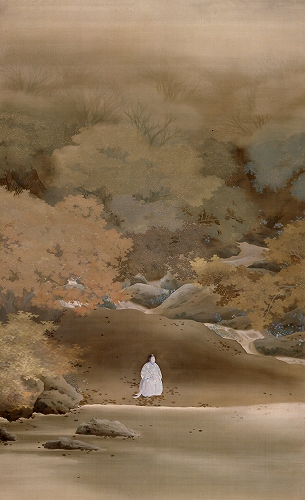The painting, a tall and narrow piece measuring three inches wide by five inches tall, appears to be a subdued and contemplative artwork, likely created with watercolors. It depicts an Asian landscape featuring a serene forest scene on a mountainside shrouded in mist. The color palette is dominated by muted, natural tones such as browns, grays, beiges, olive greens, and subtle pinkish tans, which give the piece a somewhat dreary yet harmonious feel.

In the foreground, a lone figure wearing a detailed, bulbous white robe stands or sits on a sandy or earthen bank at the bottom of a gentle slope. Their presence is both central and captivating amid the tranquil setting. The surrounding trees are painted impressionistically, with fluffy, cloud-like foliage that captures the eye, while some stray, leafless branches reach out sporadically. The trees also exhibit some crisp edges that contrast with their overall soft portrayal.

The background features rocks and a grove of bushes that blend seamlessly into the misty atmosphere, with the sky maintaining the painting's overarching earthy tones. Scattered leaves lie across the ground, adding to the scene's organic texture. Notably, the artwork lacks any text, date, or artist signature, leaving the viewer to fully immerse in its quiet natural beauty.